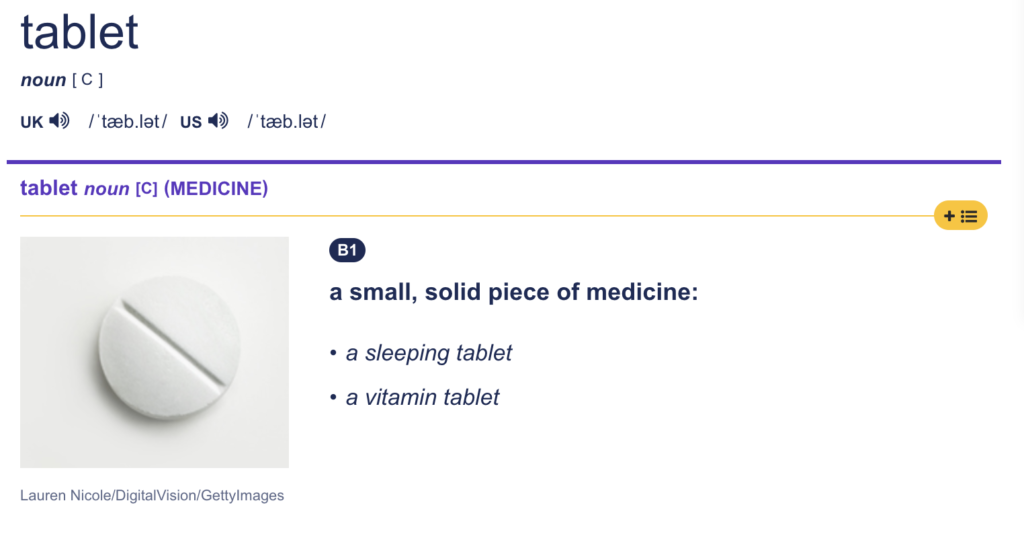The image features a pharmaceutical tablet, accompanied by several informational elements. The term "tablet" is written in lowercase and identified as a noun. Next to the word, there are speaker icons that allow you to hear the UK and US pronunciations of the word. 

In the center of the image is a picture of a standard tablet: a small, circular, white object with a bisecting line down the middle, framed by a white rectangle. To the right of the image, there is additional explanatory text. The text contains the heading "B1" inside an oval-shaped blue symbol. Below this, a definition is provided: "a small solid piece of medicine, for example, a sleeping tablet or a vitamin tablet". This descriptive information offers examples of common uses for a tablet and visually represents its appearance. 

Overall, the caption provides a comprehensive explanation of the tablet, including pronunciation, visual identification, and typical applications.